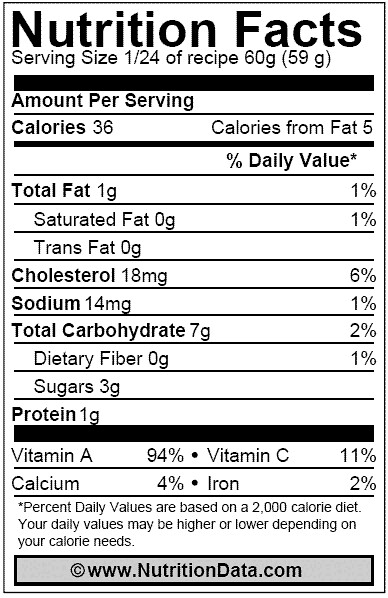This image showcases a Nutrition Facts panel with a clean, white background and black text. Dominating the top of the panel, "Nutrition Facts" is prominently displayed in large, bold letters. Just beneath this, the serving size is detailed: "Serving size 1/24th of recipe (60 grams)," followed by "(59 grams)" in parentheses. A thick, black rectangular divider bar separates this section from the nutritional information below. Proceeding downward, the panel lists "Amount per serving: Calories 36, Calories from fat 5." Additional nutritional details continue beneath this. At the very bottom of the panel, a long gray rectangle with a fine black border encloses the text "Copyright www.nutritiondata.com," prominently centered within the rectangle.